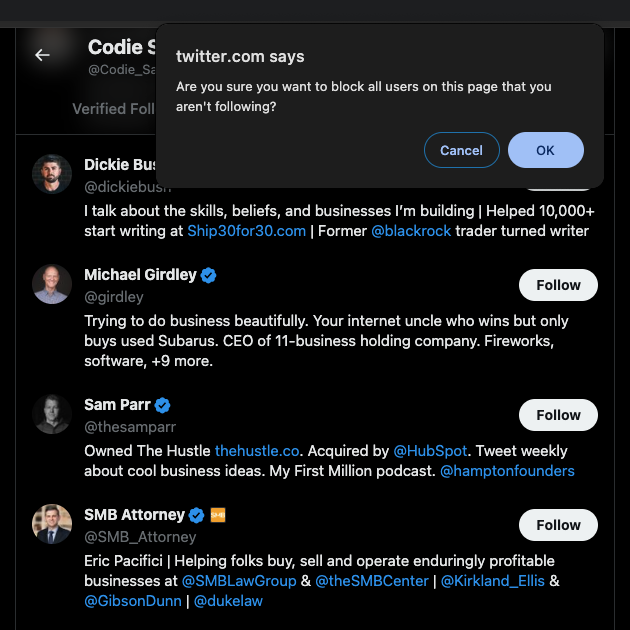**Screenshot from Twitter Interface**

In this Twitter screenshot, we observe the profile of Cody S (handle: @Cody_S), though the full handle is partially obscured. Cody S is a verified user. A pop-up window prompts, "Are you sure you want to block all users on this page that you aren't following?" with two action buttons at the bottom: a grey "Cancel" button on the left and a blue "OK" button on the right.

Below the pop-up, four accounts are listed, each with a "Follow" button on the far right:

1. **Dickey Bush:** 
   - Bio: "I talk about skills, beliefs, and businesses I'm building. Helped 10,000+ start writing at ship30for30.com. Former Blackrock trader turned writer."

2. **Michael Girdley:**
   - Bio: "Trying to do business beautifully. Your internet uncle who wins but only buys you Subarus. CEO of 11 business holding companies including fireworks and software ventures."

3. **Sam Parr:**
   - Bio: "On The Hustle at thehustle.co (acquired by HubSpot). Tweets weekly about cool business ideas. Co-host of 'My First Million' podcast. Founder of Hampton."

4. **SMB Attorney (Eric Pacifici):**
   - Bio: "Helping folks buy, sell, and operate enduring profitable businesses at SMB Law Group and SMB Center. Professional associations include Kirkland & Ellis, Gibson Dunn, and Duke Law alumni."

The profile descriptions reveal their professional backgrounds and areas of expertise, giving insight into their personal brands and contributions to their fields.